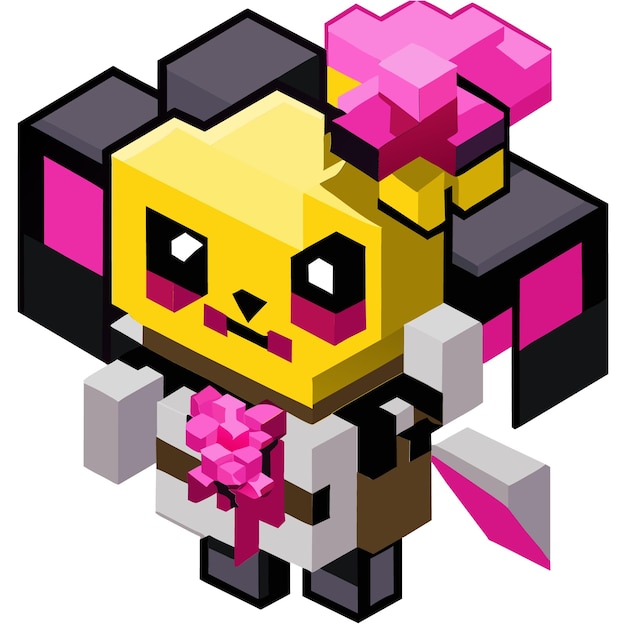This is a detailed, pixelated 3D image of a small fantasy creature, created with a blocky, abstract, almost Lego-like style. The creature has a bright yellow face with black eyes outlined by burgundy or red below them. A triangular nose sits above a straight black line mouth, accented by single red pixels at the corners. On top of its head is either a pink ribbon bow or a flower, adding to the ambiguity of whether the creature is female or not. Surrounding its head is some black pixelation that could represent hair or possibly ears. The creature's body is silver and brown, adorned with a pink bow at the front, suggesting it might represent a gift or a dress-like outfit. In its hand, it holds a pink and silver sword, while standing on solid black feet. The background is plain white, emphasizing the vibrant colors and intricate details of the character.